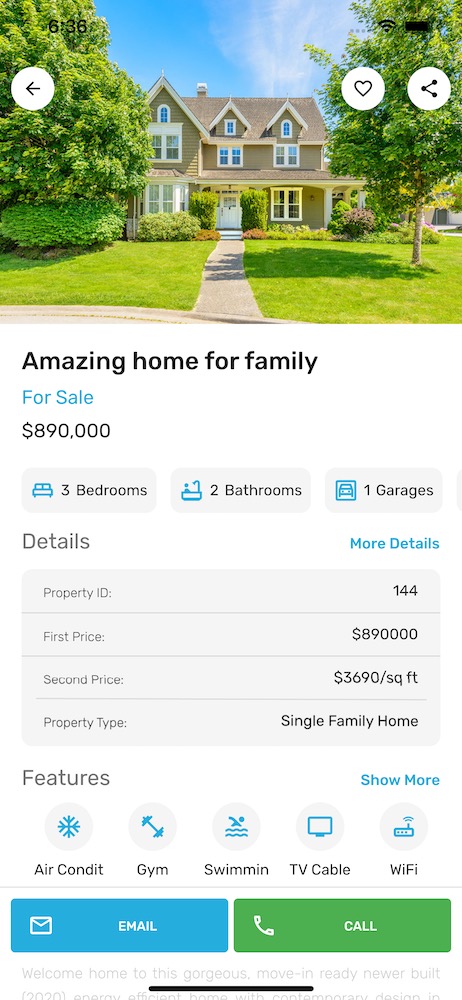This image is a color screenshot from a real estate app or website, displaying a listing for a classic American-style detached home. The property is portrayed as a three-story house, featuring a charming wooden exterior with brown paint and white shutters. The home is characterized by three prominent triangular roofs and is surrounded by a large, well-maintained lawn with a pathway leading up to the front door, framed by trees.

The listing headline beneath the photo highlights the home as "Amazing Home for Family for Sale" with a price tag of $890,000. The house boasts three bedrooms, two bathrooms, and a garage. Additional information provided includes the property ID number 144 and a price per square foot of $3,690. The home is identified as a single-family residence.

Key features of the property include air conditioning, a gym, a swimming pool, TV cable, and Wi-Fi. At the bottom of the listing, users are given the option to either email or call for more information, via a blue button for emailing and a green button for calling.